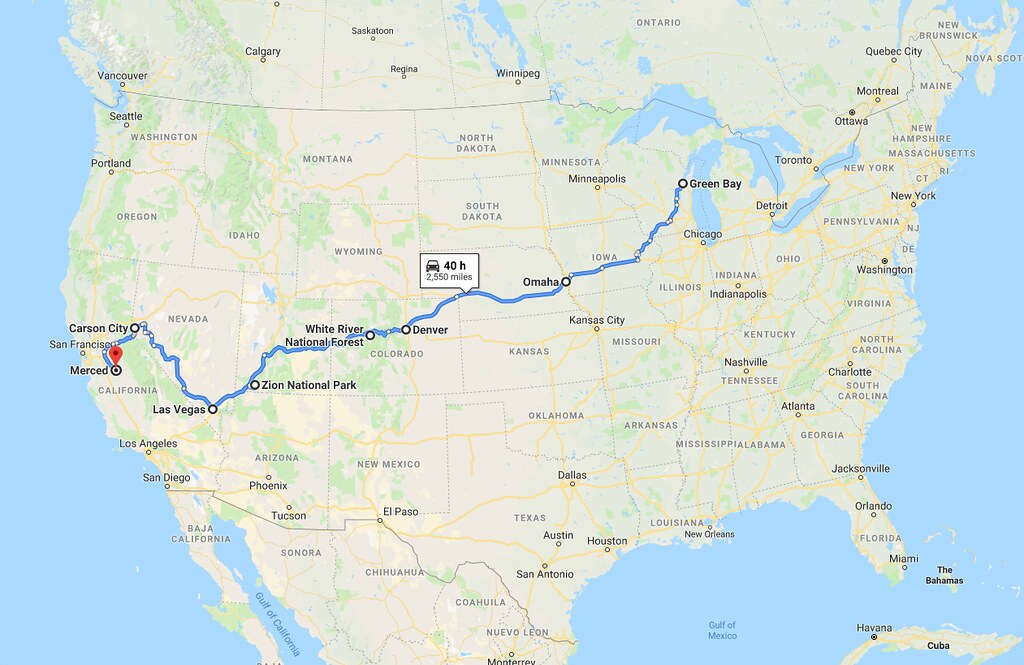The image portrays a map of the United States set against a blue background, featuring a prominent blue line that represents a cross-country route. This journey begins in Green Bay, Wisconsin, and extends all the way to Merced, California, and San Francisco. Along this extensive route, key cities and landmarks are highlighted, showcasing a variety of destinations one would encounter. The journey is marked with a notation indicating "40 hours," particularly between Omaha, Nebraska, and Denver, Colorado. The route traverses several notable cities including Green Bay, Omaha, and Denver, as well as significant natural landmarks such as the White River National Forest and Zion National Park. Further along, the path passes through vibrant locations like Las Vegas and Carson City, before reaching its final points in San Francisco and Merced, California. This detailed trajectory essentially spans across the entirety of the United States, depicting a comprehensive east-to-west travel route.